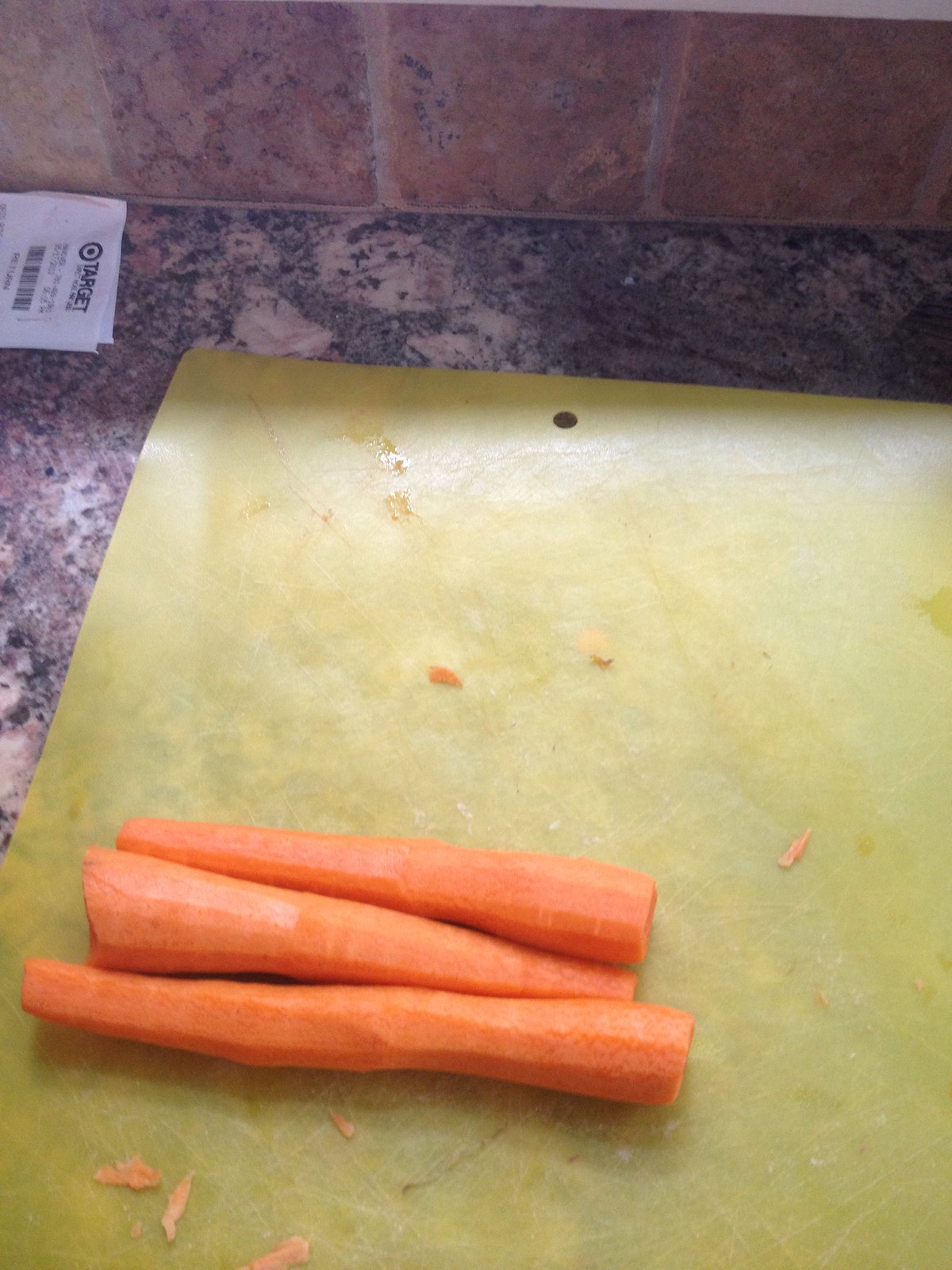This image features a granite countertop with a pink-tinged granite backsplash. Positioned in the upper left corner of the countertop is a Target receipt. Prominently displayed on the off-white, flexible cutting board are three whole, peeled carrots arranged with alternating orientations: the bottom carrot points left, the middle carrot points right, and the top carrot points left again. The cutting board has a yellow tint, suggesting it was designed that way, and includes a hole for hanging. Scattered on the board are some carrot shavings. The background includes a portion of a wall with a faux brick design, adding to the kitchen setting's detail.